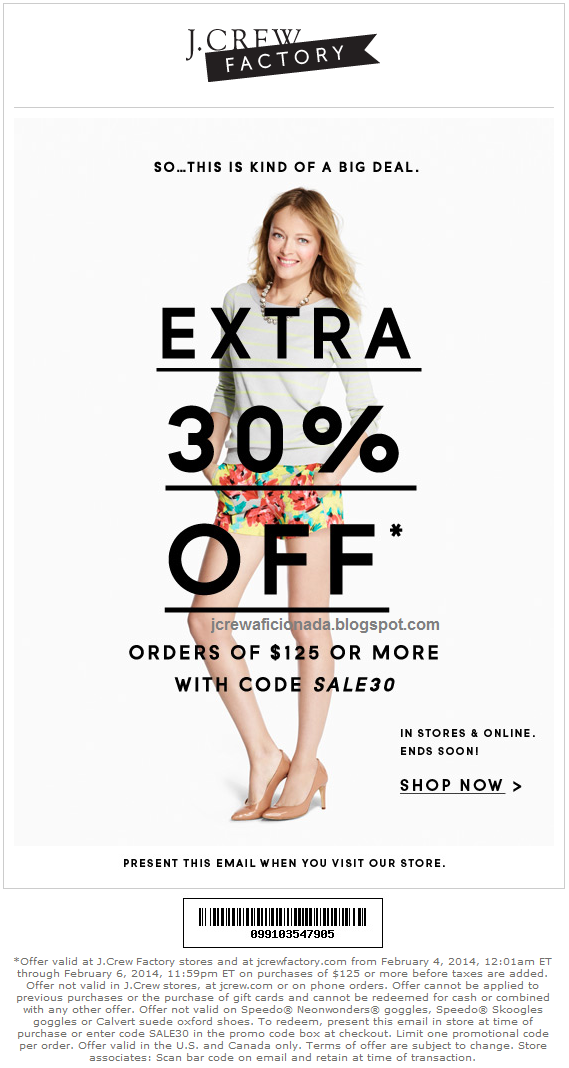Here's a refined and detailed caption for the described image:

---

The image showcases a promotional webpage from J.Crew Factory. Set against a white background, the top of the page prominently features the "J.CREW" name in capital letters, with a "FACTORY" banner, indicative of the brand's logo. Below this header, a horizontal line delineates the main content area.

In the body of the page, bold text reads "So... This is kind of a big deal." A center-aligned photo captures a stylish woman adorned with a necklace, a shirt, shorts, and heels. Overlaid on the image, starting at her neck, bold text announces "EXTRA 30% OFF."

Further promotional details are listed below, including the URL "jc.rew.officio.nada.blogspot.com." The conditions of the offer specify, "30% off orders of $125 or more. Use code SALE30 in-store and online. Ends soon. Shop Now!" The call-to-action link is clickable, and below it is a statement instructing customers to present the email during their store visit.

A barcode, numbered 099103547905, is displayed, accompanied by fine print that details the terms of the offer. It states the promotion is valid at J.Crew Factory stores and online at J.CrewFactory.com, from 12:01 AM ET on February 4, 2014, through 11:59 PM ET on February 6, 2014, for purchases of $125 or more before taxes. The offer is not valid at standard J.Crew stores, J.Crew.com, or for phone orders. Restrictions apply, including exclusions for previous purchases, gift card purchases, and specific products like Speedo Neon Wonders Goggles and Calvert Suede Oxford shoes. Customers are advised to present the email in-store or enter the code "SALE30" during online checkout. The promotion is limited to one code per order and is valid only in the US and Canada. Terms are subject to change, and store associates must scan and retain the email barcode at the time of the transaction.

---